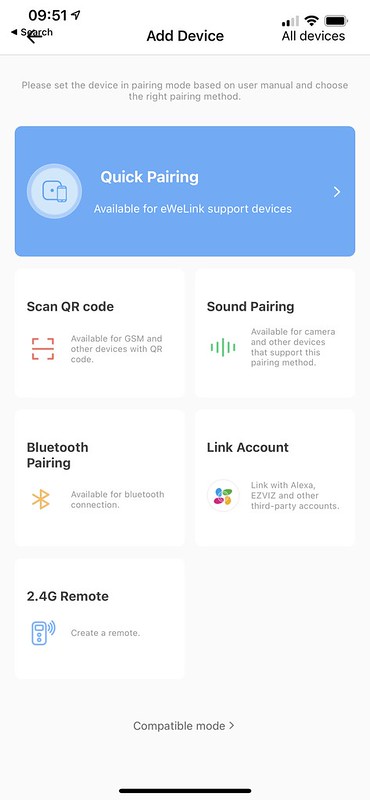This image captures a screenshot of a web page viewed on a cell phone. Across the top of the screen, the time is displayed as 9:51, and the status bar shows icons for battery life, Wi-Fi, and signal strength. Below the status bar, there is a search bar partially obscured by a hand-drawn black arrow, likely added with a marker tool, making the text difficult to read. 

Just underneath, the screen shows an option labeled "Add Device," and to the right, "All Devices." Further down, a section titled "Quick Pairing" is visible, accompanied by a clickable blue button labeled "Available for eWeLink-supported devices." 

The lower section of the page features five interactive squares or tiles. The top left tile reads "Scan QR Code," and next to it, the top right tile says "Sound Pairing." In the row below, the bottom left tile is labeled "Bluetooth Pairing," while the one to its right says "Link Account." Finally, the bottom tile reads "2.4G Remote."